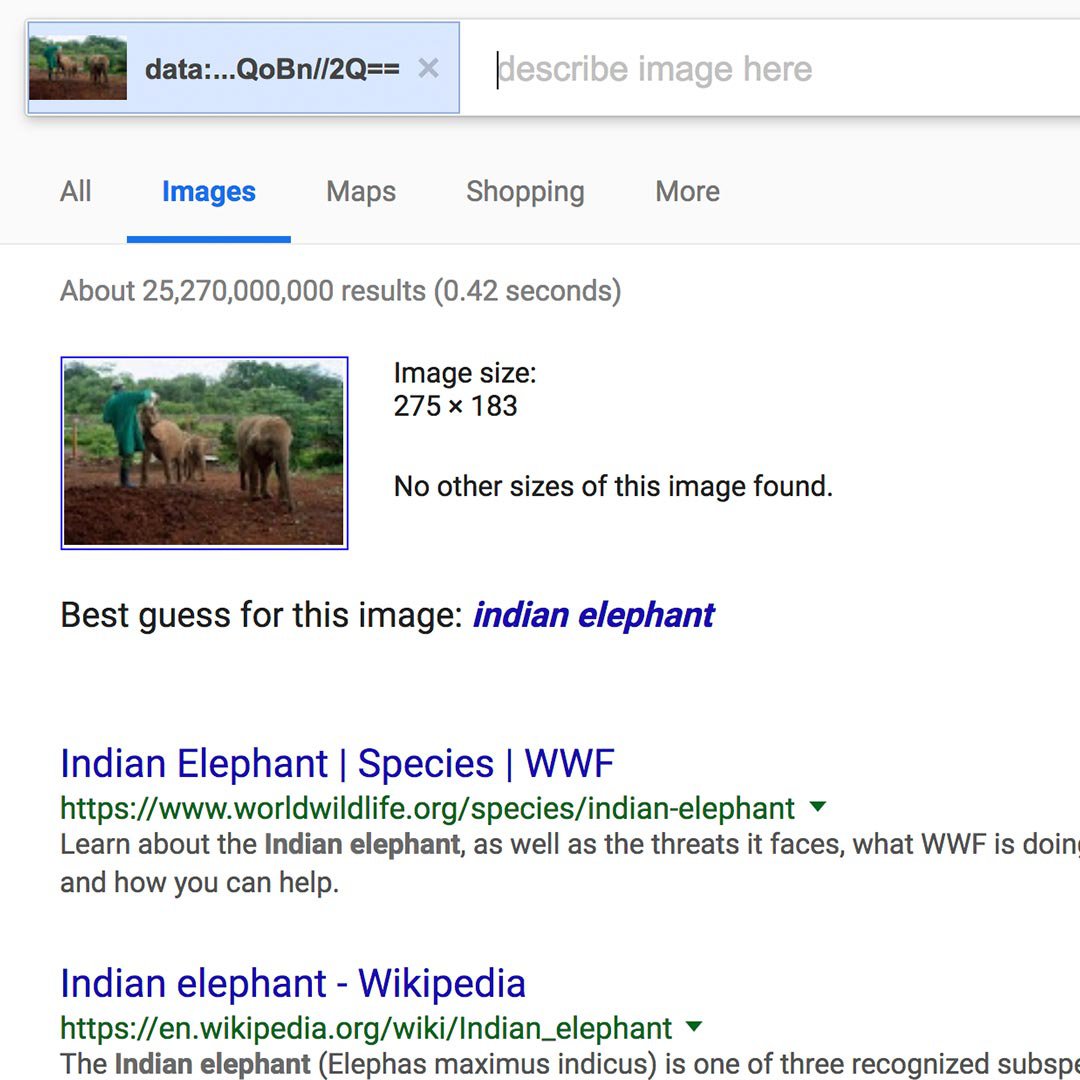This image appears to be a screenshot taken from a computer screen. At the very top, there is a blue toolbar with a small picture in the upper left-hand corner, depicting some animals outdoors, potentially cows. Next to the image, there is a text string that reads "data QOBN // TQ ==." To the right of the toolbar is a white search bar that says "describe image here."

Below the toolbar, there are several tabs labeled "All," "Images," "Maps," "Shopping," and "More." The "Images" tab is highlighted, indicating that image search results are displayed. The search results note that there are approximately 25,270,000,000 results.

Below this, the previously mentioned image of animals, which resemble cows, is shown once again. To the right of this image, there is information indicating the image size as 275 by 183 pixels and notes that no other sizes of this image have been found.

Further down, there is a section titled "Best guess for this image," identifying the image as that of an "Indian elephant." Listed below are two website links related to Indian elephants. The first link points to the WWF website with the text "Indian elephant species - WWF," followed by the URL "worldwildlife.org/species/indian-elephant." The second link directs to a Wikipedia page with the text "Indian elephant - Wikipedia," followed by the URL "wikipedia.org/wiki/Indian_elephant."